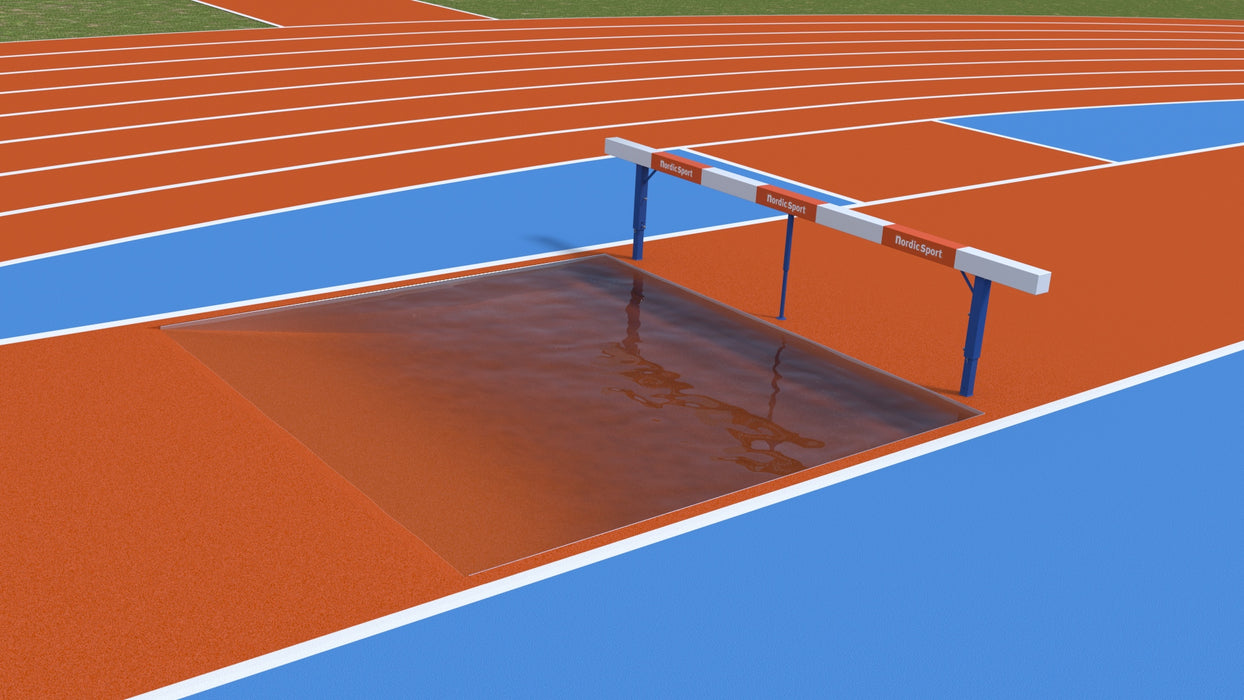This image depicts what appears to be a high school or competition track field featuring a steeplechase hurdle and water pit. The track is predominantly orange with defined white lane markings and includes prominent blue areas – one in the bottom left corner, another to the right, and a third one in the center. The hurdle, marked with "Nordic sport," spans the track just before a square water pit, commonly used in steeplechase events. Additional details include green grass patches visible in the background, as well as a defined running path potentially for high jump activities. The surroundings of the track break up the overall red-orange color with these distinct blue and green elements.